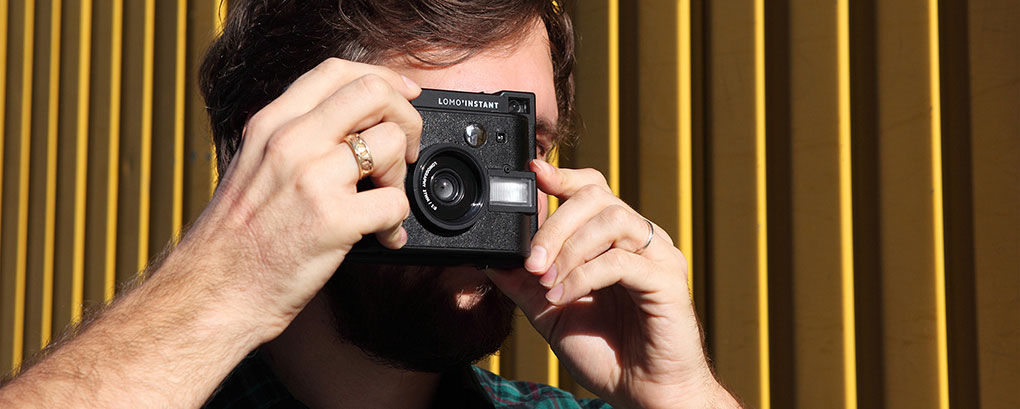This is a detailed image of a Caucasian man with dark brown, slightly swoopy hair and a possible beard, taking a photo with a black Lomo Instant camera. He is holding the camera up to his eye with both hands. Notably, he is wearing a gold wedding ring on his left hand and a silver band on his right ring finger. His attire includes a green and black checkered shirt, partially visible from his left shoulder. The background features a series of vertical yellow slats of varying spacing, creating an interesting geometric pattern. The man appears well-lit from the front, casting shadows behind him.